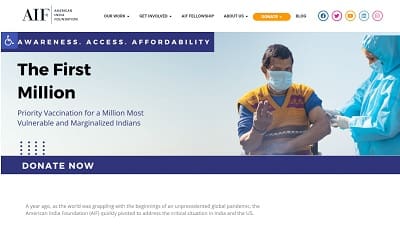This screenshot captures the homepage of the AIF (American India Foundation) website. In the upper left corner, the AIF logo prominently appears against a white background that spans the website’s menu bar, extending across the top of the image. Due to the distant view, the exact details of the menu options are unclear.

Below the menu bar, a banner is displayed. On the upper left side of this banner, there is a symbol indicating accessibility for handicapped individuals, emphasizing inclusivity. To the right of this icon, there are the words "Awareness. Access. Affordability." inscribed in a blue horizontal band, underscoring the foundation's primary missions.

Underneath this, the main text reads "The First Million" followed by smaller text that states, "Priority vaccination for a million most vulnerable and marginalized Indians." This concise message highlights the AIF's campaign focus on prioritizing COVID-19 vaccinations for at-risk populations.

On the right side of the banner, there is a visual of two individuals, where one person is administering a vaccine to the other, reinforcing the message of the campaign.